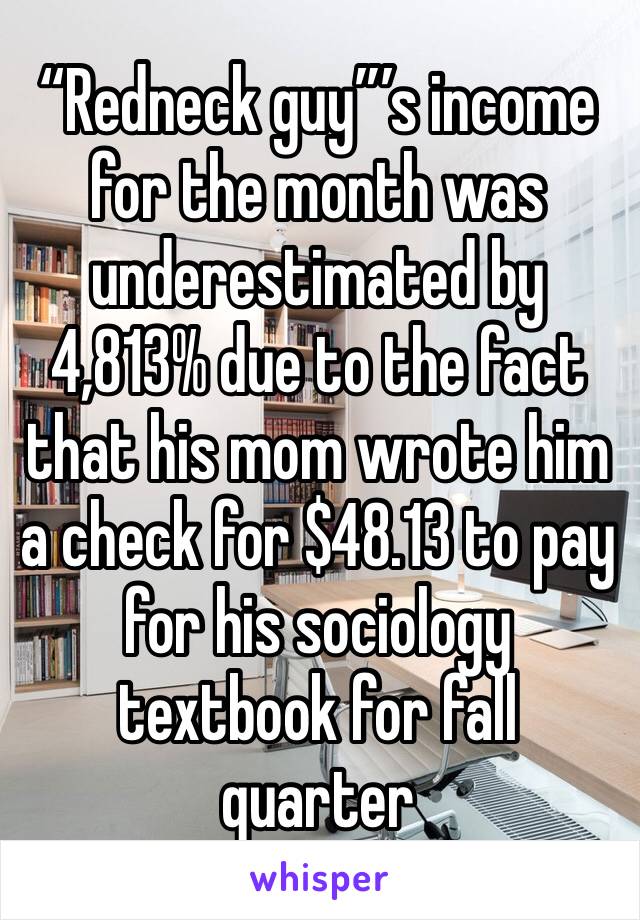The image appears to be a humorous meme intended for social media, featuring bold, white text with a black outline that occupies most of the screen. The text reads, "Redneck Guy's income for the month was underestimated by 4,813% due to the fact that his mom wrote him a check for $48.13 to pay for a sociology textbook for fall quarter." Below this main text, in a white banner, the word "Whisper" is prominently displayed in purple. The background depicts a home office with white walls, white curtains, and white window sills. There are shelves filled with various books on the left side of the image and a wooden desk with a black computer monitor and an office chair in the bottom right corner. The overall scene suggests a casual, somewhat cluttered office space, characterized by colors such as white, gray, black, red, orange, purple, green, silver, and tan.